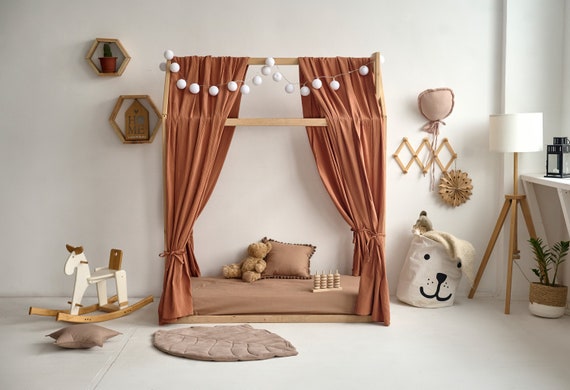This detailed photograph captures the interior of a bright, white-walled child's bedroom. Central to the scene is a floor-level bed or cushion draped with a pink sheet, complemented by a matching pink pillow. Nestled on the bed is a tan-colored teddy bear. Suspended above the bed are wooden bars forming a canopy adorned with light brown sheets and decorative blue balls that may serve as lights or simple ornaments. To the far left, a white and brown wooden rocking horse stands out. Also visible on the left is a decorative brown star-shaped pillow. The floor, which is white tile, features a toy characterized by small stackable items. To the right, there is a unique clothing hamper styled with a white dog's face, complete with eyes and a nose. Natural light illuminates the space, highlighting the serene and playful atmosphere of the room.